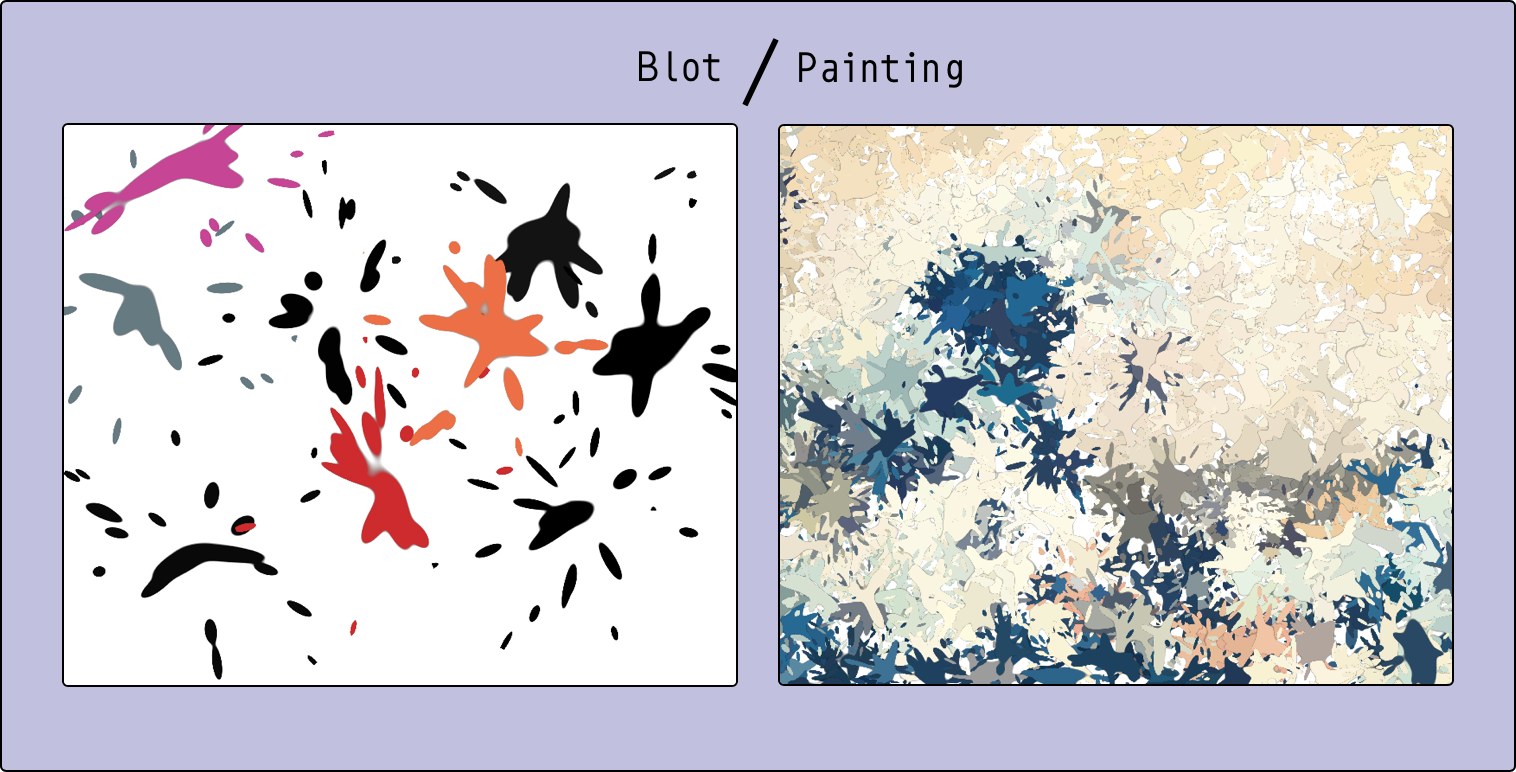The image appears to be part of an educational series, consisting of two professionally photographed pictures placed side by side, framed by a purple background typical of PowerPoint presentations. The duo is enclosed within a blue border with the caption "blot/painting" displayed at the top.

On the left, the image showcases a white square backdrop adorned with variously colored ink or paint blots. The colors include black, white, greenish-blue, orange, red, raspberry pink, purple, gray, beige, and taupe. These splashes have a radial pattern, as if liquid was thrown onto the surface, creating a central blot with smaller surrounding splashes.

The image on the right is a more complex representation, resembling a painting with overlapping splotches of color. Dominated by shades of blue, tan, taupe, and gray, this picture also includes brown and highlights of lighter pink and off-white hues. The arrangement of colors suggests a leafy pattern, contributing to a sophisticated visual impression compared to the first image.

Overall, the presentation aims to contrast the simple technique of blotting with the layered complexity of painting, serving an educational purpose.